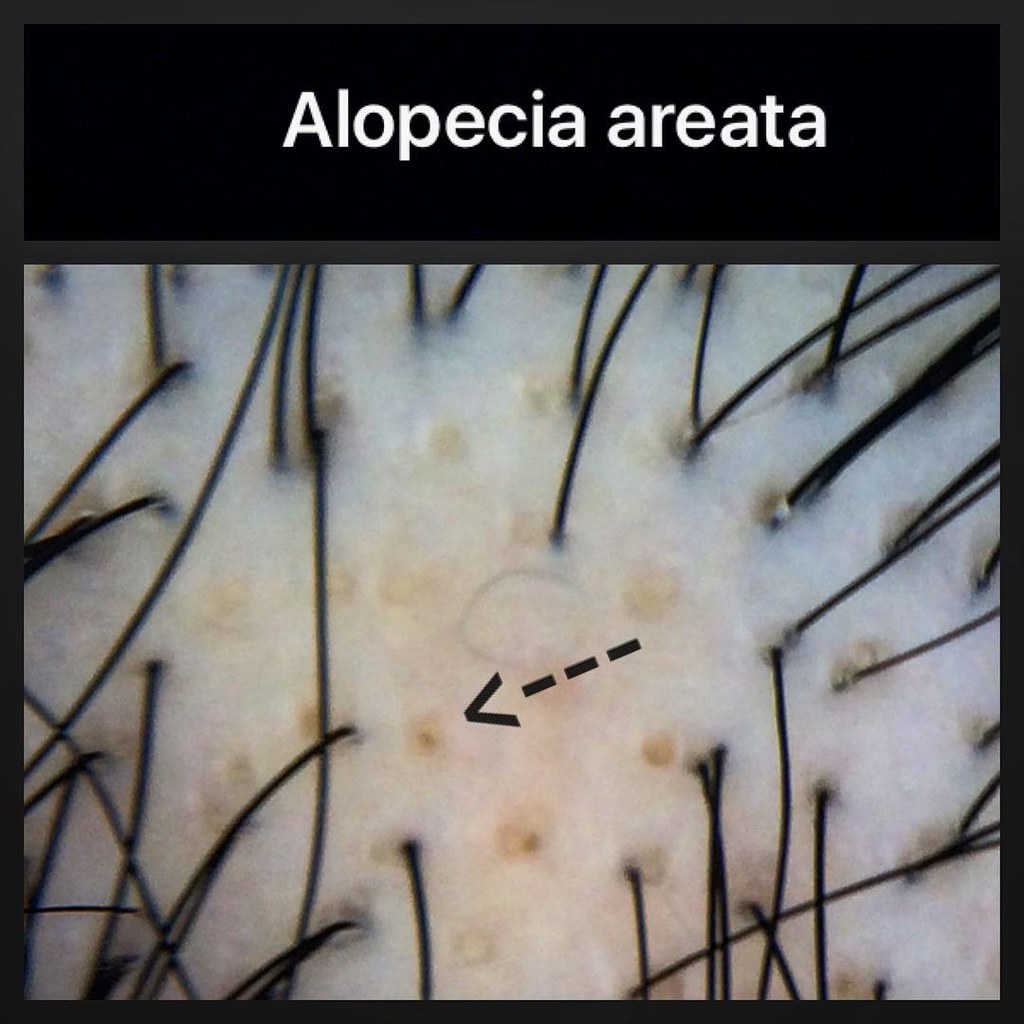The image is a detailed infographic about Alopecia Areata, framed within a sleek black border. At the top of the image, "Alopecia Areata" is prominently displayed in white text on a black rectangular banner. Below this header, the main graphic presents an extreme close-up of pale skin, dotted with numerous hair follicles. Some follicles are growing sparse black hairs, while a prominent black dotted arrow points to one specific hair follicle, which appears empty, illustrating the condition's effect on hair growth. The entire scene is akin to a zoomed-in view of a scalp, emphasizing the areas where hair is sparse or absent due to alopecia. The simplicity of the layout, with its clear focus on one highlighted pore, effectively communicates the nature of this hair-loss condition.